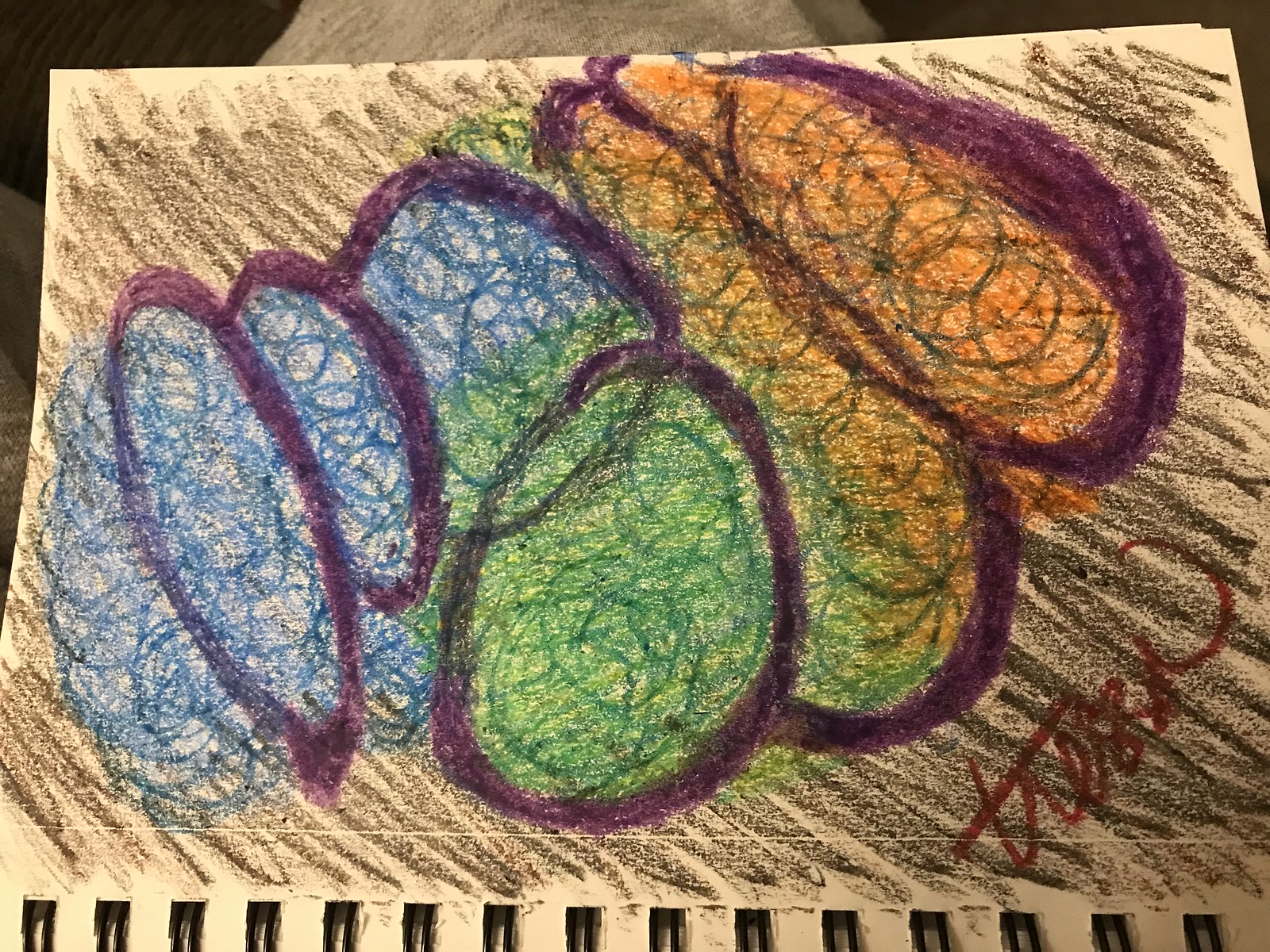This color photograph captures a detailed and abstract drawing on white paper within a spiral-bound notebook, evident by the black bindings along the bottom edge of the page. The artwork features a central arrangement of spheres and elongated shapes, perhaps resembling an abstract still life, with various vibrant colors filling each form — shades of blue, green, orange, and yellow. The shapes are outlined prominently in deep plum and purple hues, with swirls and scribbles enhancing their texture and sense of movement. Overlapping these colorful elements are numerous purple circles. The remaining white space is energetically filled with black crayon scribbles. At the bottom right corner of the image, a signature in red crayon, possibly reading "Teresa," adds a touch of personal authenticity to the piece. The drawing is set against a darker backdrop, with black and gray elements visible behind the paper, contributing to the image's layered composition.